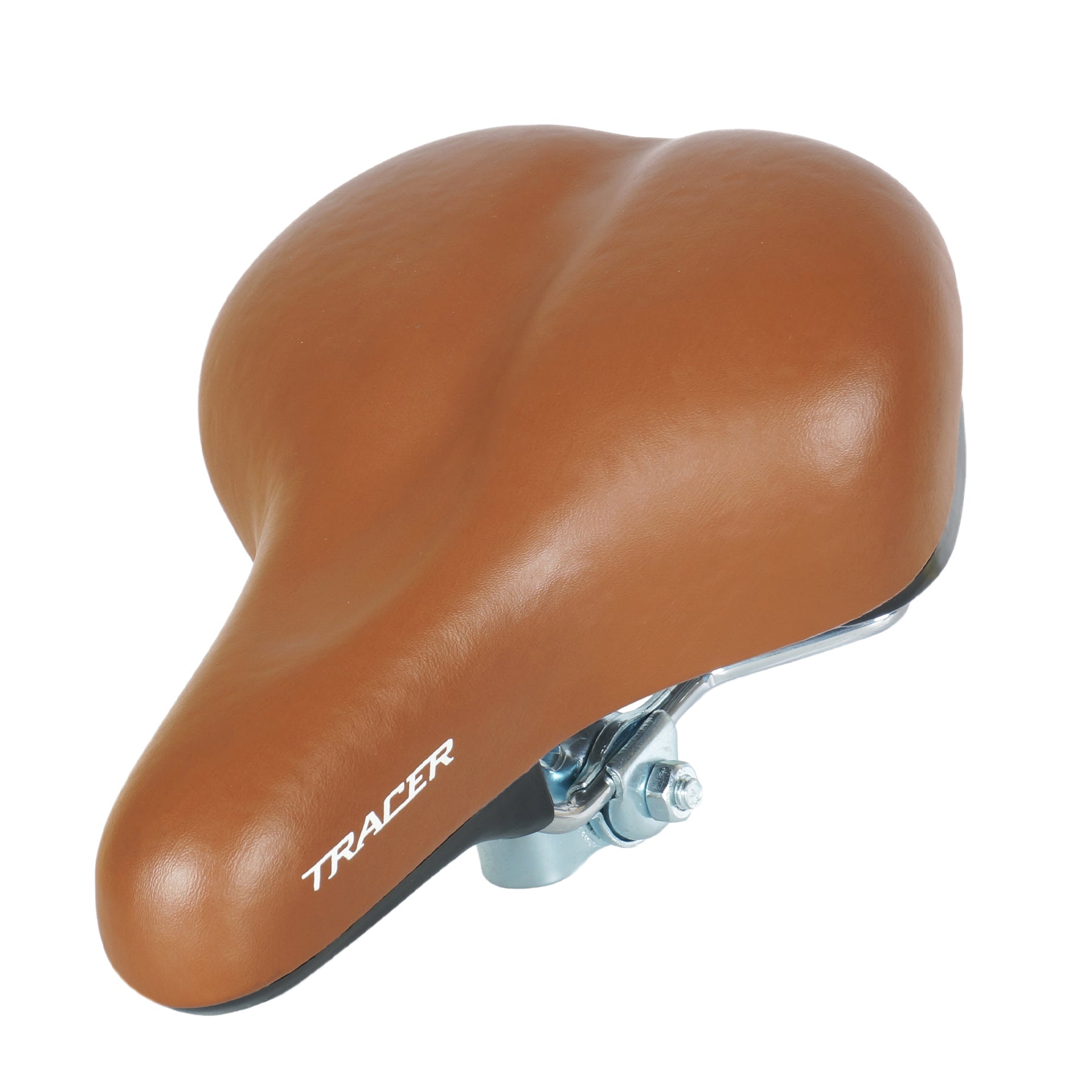This image showcases a professionally lit and photographed bicycle seat against a plain white background, likely intended for a catalog or a website. The seat is covered in medium brown material that resembles leather, possibly a high-quality facsimile. The seat features a distinct shape: a wider, rounded back for seating that tapers into a narrower, elongated section toward the front. The brand name "Tracer" is prominently displayed in all caps white block lettering, which is more of a graphic design style with the letters joined together on the front right side of the seat's horn. Below the brown seat cover, there is a black base, possibly made of hard plastic, and beneath that, a visible metallic mechanical bracket designed for attachment. This bracket includes screws and bolt inserts for secure mounting. The detailed craftsmanship and high-resolution detail indicate its likely use in promotional material.